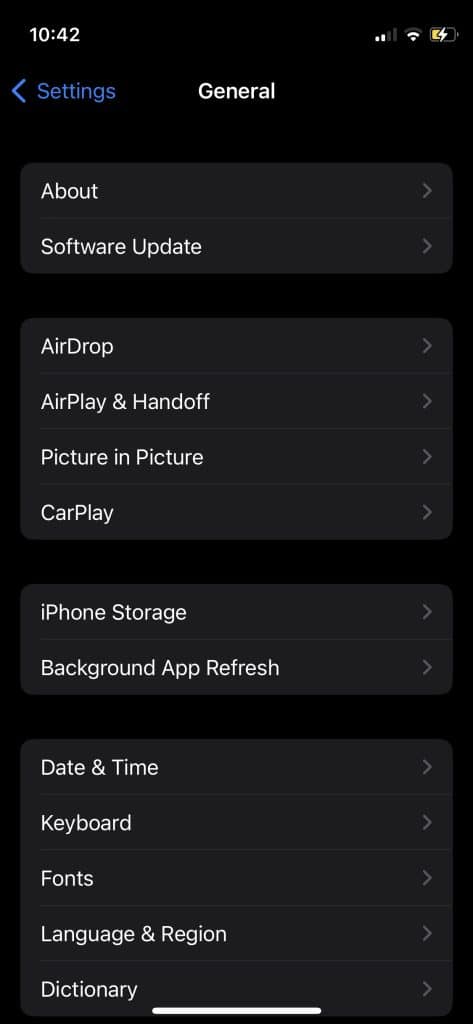The image showcases a screenshot of an iPhone displaying the settings menu, set against a dark theme. At the top of the screen, the time is shown as 10:42 on the left, while the network signal strength is indicated as 2 out of 4 bars, and the Wi-Fi signal strength as 2 out of 3 bars on the right. The battery icon shows that the device is currently charging.

In the main area of the screen, the settings menu includes the following options: Settings, General, About, Software Updates, AirDrop, AirPlay & Handoff, Picture in Picture, CarPlay, iPhone Storage, Background App Refresh, Date & Time, Keyboard, Fonts, Language & Region, and Dictionary. At the bottom of the image, the iPhone navigation pill is visible.

The color scheme features text in white, blue, and grey, set against the black background of the dark theme, providing a stark contrast that makes the interface elements easily readable.